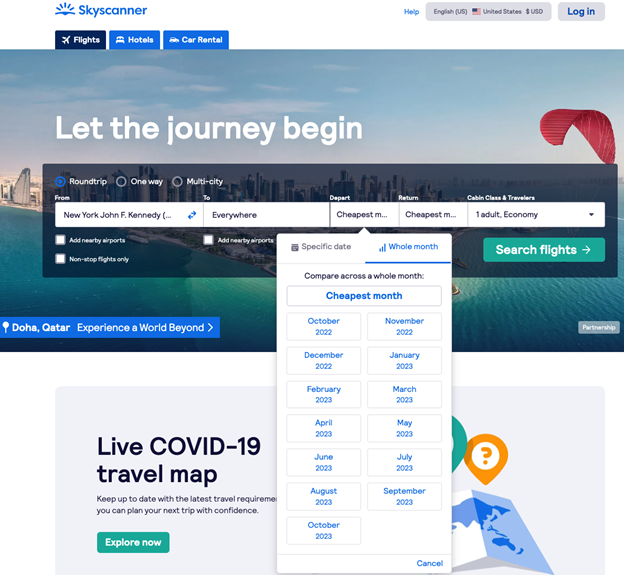**Detailed Caption:**

This is a screenshot of a webpage from the travel website, Skyscanner. The website features the Skyscanner logo at the top, which consists of a blue icon resembling the rays of a sun rising over a horizon, paired with the word "Skyscanner" in blue text. Below the logo are three clickable tabs labeled "Flights," "Hotels," and "Car Rental." The "Flights" tab is currently selected.

Dominating the main section of the page is a large, vibrant background image showing an aerial view of Sydney Harbour, Australia, with sparkling blue and green waters against a sprawling cityscape. However, a prominent pop-up prompt partially obscures the iconic Sydney Opera House in the background. Overlaid on this scenic picture are various interactive boxes for users to input their departure and destination locations, as well as other flight booking details. The overall layout and design indicate that the purpose of the website is to facilitate flight bookings.